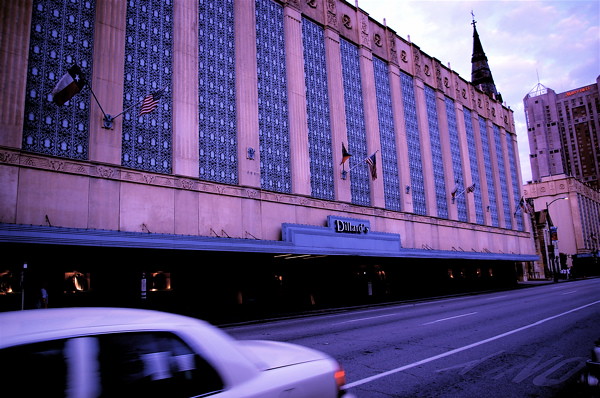A photo captures a historic Dillard's department store building from across the street, viewed at an angle from the left side. This large, slightly weathered building boasts classic architecture, suggesting it may have been repurposed from an old theater or hotel. An array of flags, including the American and Puerto Rican flags, adorns its roof. To the right, the top of a cathedral-style building with a cross is visible, while adjacent to Dillard's lies another department store building. In the distant background on the right, a Marriott hotel stands prominently. A whitish gray car can be glimpsed in the lower left corner, indicative of the photo being taken from a roadway or perhaps from within another vehicle.